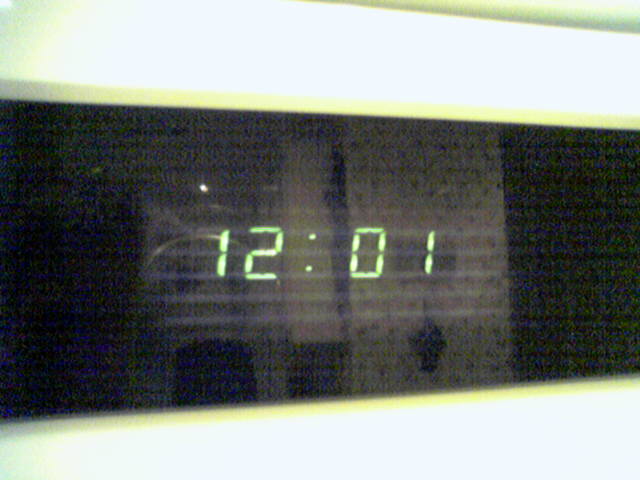This is a blurred, horizontal photograph of an LED clock with a digital display. The time shown is 12:01, illuminated in a bright, neon green against a black and blue background. The clock face is framed by a pale yellow border, set against a broader white backdrop. There appears to be an indistinct reflection on the display—possibly resembling receipts or strips with writing—though its details are unclear. The overall photo quality is not very high.